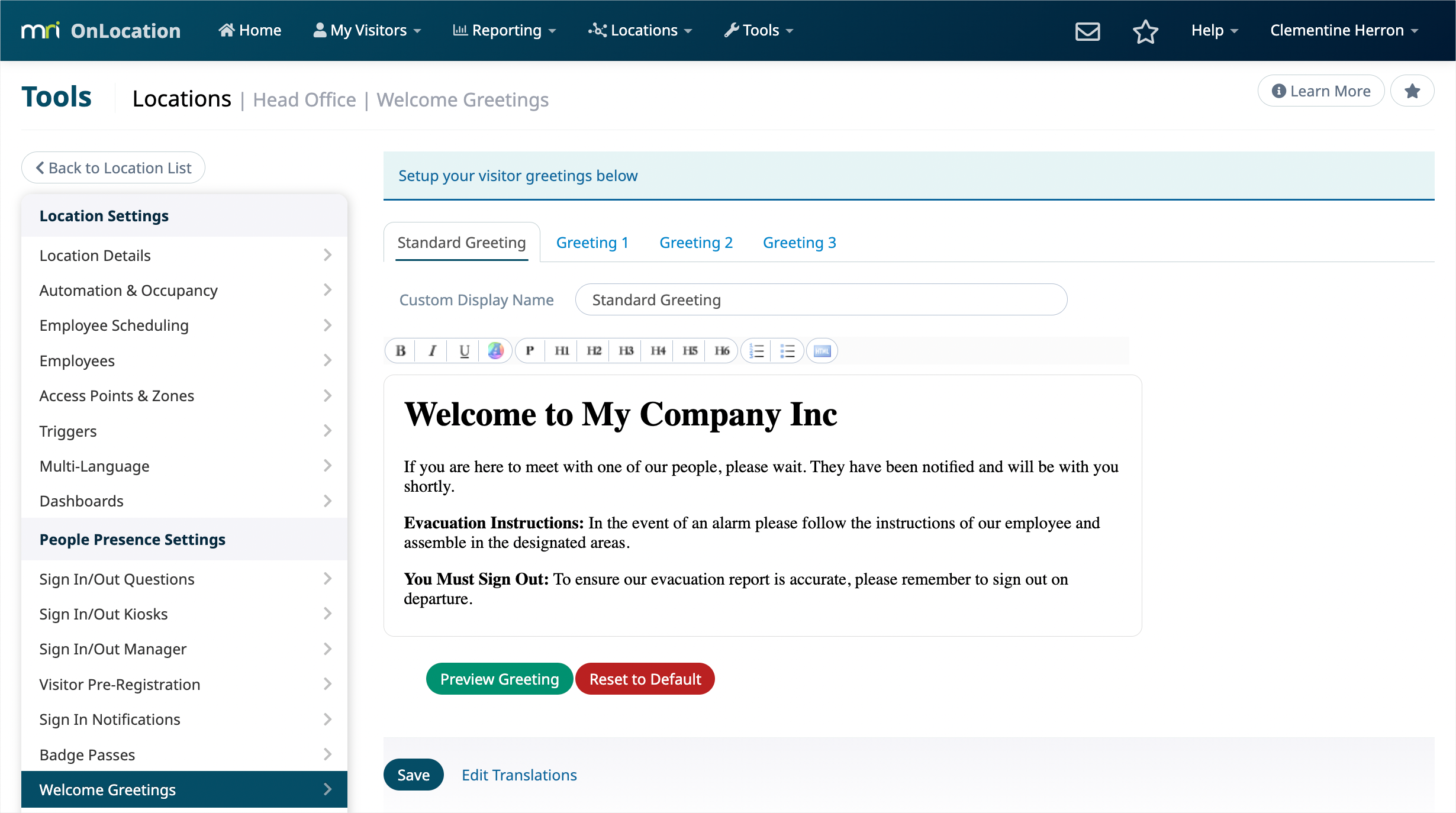The image depicts a detailed view of a website interface with a sleek design. At the top is a dark blue banner featuring the text "MRI," where the 'R' and the dot above the 'I' are highlighted in green. Adjacent to this, "OnLocation" is written as a single word with capital letters 'O' and 'L'. 

The navigation bar includes the following options, each with dropdown menus: Home, My Visitors, Reporting, Locations, and Tools. On the right side of this bar, there are icons for an envelope, a star, and a help section with a dropdown menu. The user's name, "Clementine Heron," is also displayed with a dropdown menu.

Below the banner, the background shifts to white, and several sections are highlighted: Tools, Location, Head Office, and Welcome Greetings. On the right, there are links to "Learn More" and "Back to Location List."

A sidebar on the left provides an extensive menu with the options: Location Settings, Location Details, Automation and Occupancy, Employee Scheduling, Employees, Access Points and Zones, Triggers, Multi-Language, Dashboards, and People Presence Settings in bold text.

Further down, the options expand to include Sign In/Out Questions, Sign In/Out Kiosks, Sign In/Out Manager, Visitor Pre-Registration, Sign In Notifications, Badges, and Welcome Greetings. The section titled "Set up your visitor greeting below" offers standard greeting options labeled Greeting One, Greeting Two, and Greeting Three. A sample greeting reads "Welcome to My Company, Inc." Additionally, there are instructions for evacuation and a sign-out requirement. The interface includes buttons for Preview Greeting, Reset to Default, Save, and Edit Translations.